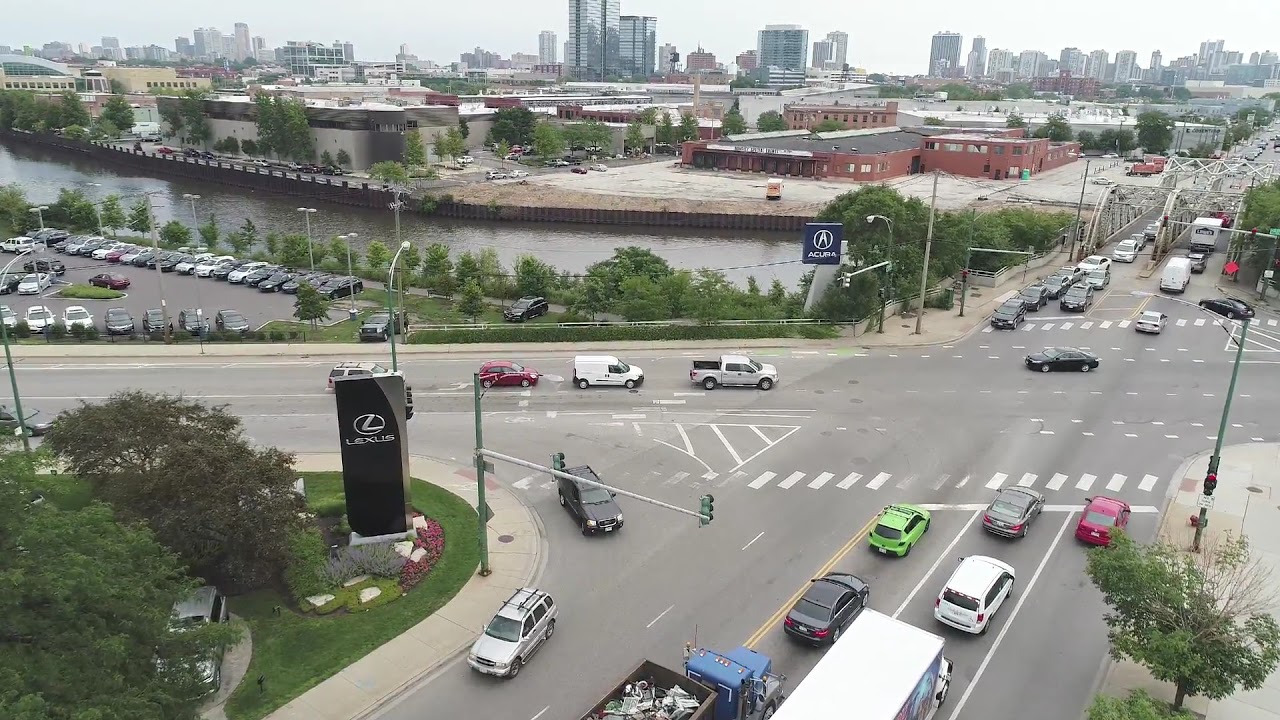The image is an overhead, high-angle shot captured either from a building or a drone, depicting a bustling urban intersection. The scene is set in a commercial area, identifiable by signs for a Lexus dealership and an Acura dealership positioned on opposite sides of the street. Multiple trees dot the area, contributing to its urban aesthetic. Amidst the intersecting streets, a small iron and steel bridge spans a river that runs horizontally through the middle of the photograph. The background features numerous buildings and industrial structures, with skyscrapers visible far off in the distance, indicating the city center. The day's gray, overcast weather casts a subdued tone over the busy street, where a mix of SUVs, sedans, and trucks are either stopped or moving through the intersection. The tallest skyscraper in the middle of the photo is entirely glass, standing prominently against other clusters of high-rises to the upper left.